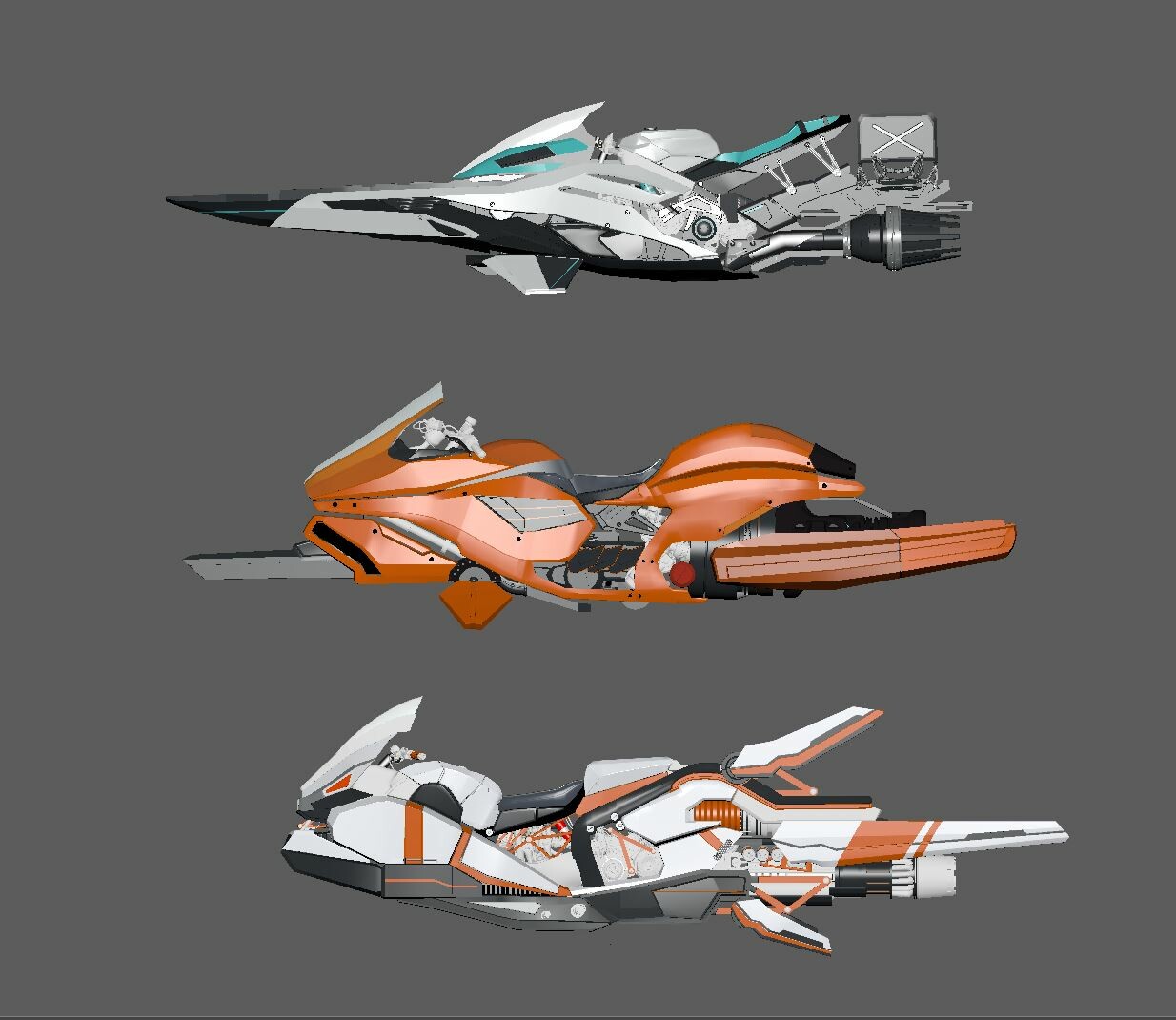The image showcases three digitally rendered, futuristic vehicles against a uniform dark gray background. These sleek, hovercraft-like designs resemble a hybrid of motorcycles, fighter jets, and jet skis, each lacking traditional wheels. The top vehicle is a streamlined, long, and narrow form, primarily gray and black with turquoise accents. It features a jet propulsion system at the rear and an elongated, boat-like front. The middle vehicle is a cantaloupe orange and gray, with a design reminiscent of a motorcycle's cockpit, possibly suggesting a rider's head emerging from behind a windscreen. This vehicle also has a horizontal beam extending outward before culminating in a jet engine. The bottom vehicle, white and gray with bold orange accents, combines elements of a Nerf gun, motorcycle, and airplane. It features fins projecting from both the top and bottom, with a sleek, flat base extending to a rear jet engine.